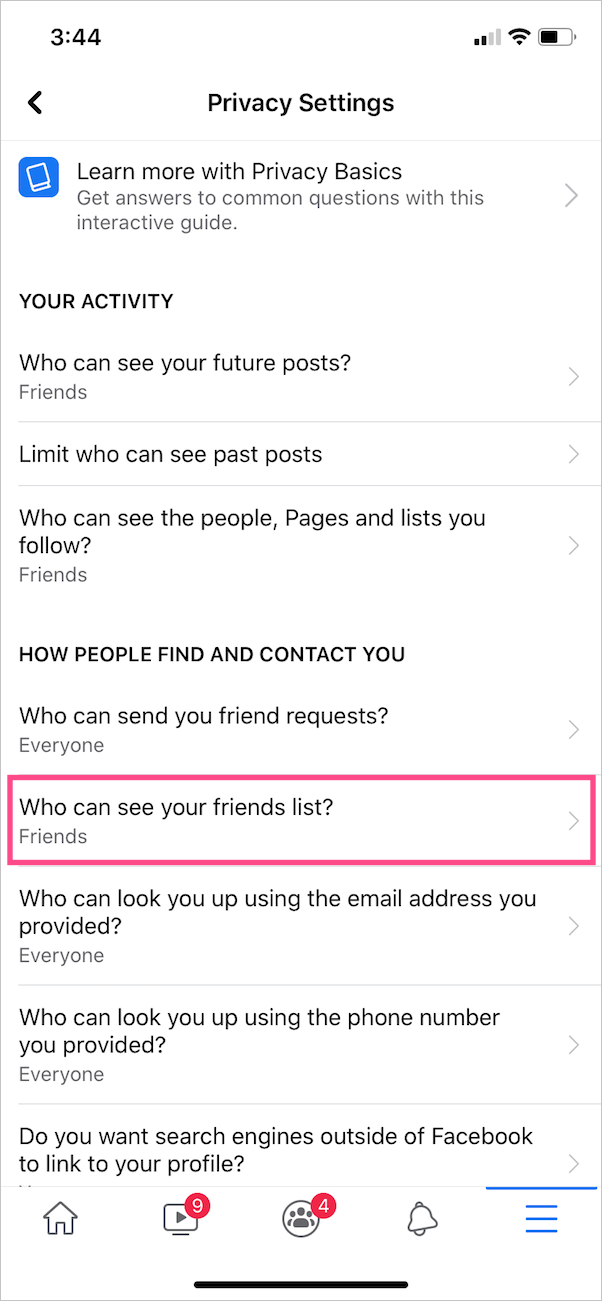This screenshot captures the privacy settings in a mobile app. The interface displays a mostly white background, with user interface elements in black font and blue accents. At the very top, the device status bar is visible, showing the time as 3:44 PM on the upper left. The upper right corner displays the mobile signal strength at two out of four bars, full Wi-Fi signal, and a half-charged battery icon.

Below the status bar, there is a heading in black font that reads "Privacy Settings." Directly under this heading is a blue square with a white book icon, accompanied by text: "Learn more with Privacy Basics. Get answers to common questions with this interactive guide," followed by a small gray arrow indicating that the guide can be opened.

Further down, several privacy options are listed, all in black font:
- "Your Activity
  - Who can see your future posts: Friends
  - Limit who can see past posts
  - Who can see the people, pages, and lists you follow: Friends"
- "How People Find and Contact You
  - Who can send you friend requests: Everyone
  - Who can see your friends list: Friends
  - Who can look you up using the email you provide: Everyone
  - Who can look you up using the phone number you provide: Everyone"
  
The final option, "Do you want search engines outside of Facebook to link to your profile," appears to be cut off in the screenshot.